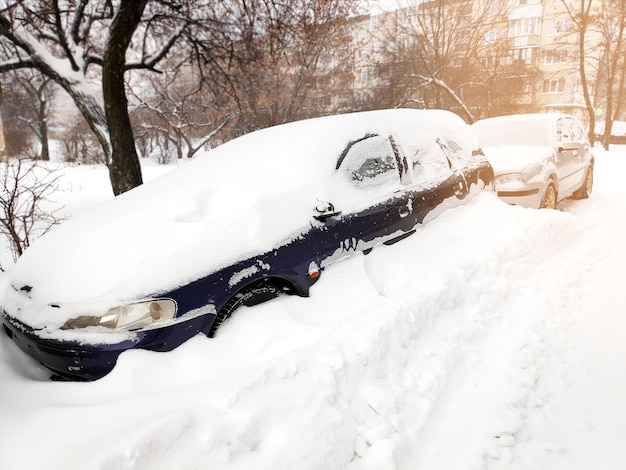This photograph captures a winter scene featuring two parked cars heavily covered in pristine, white snow. The snow blankets not only the tops but also the sides of the vehicles, rising almost to the level of the passenger and driver-side windows. Dominating the foreground is a blue estate car, possibly a Ford, deeply buried under the snow. Behind it sits an older silver car, likely a Volkswagen Golf, with a noticeably lighter snow covering.

Positioned on a slight diagonal from northeast to southwest, the cars are seen from an angle that offers a clear view of their hoods and trunks. The scene is set against the backdrop of a large, six-story apartment complex stretching across the top of the image. The apartment buildings and nearby bare trees, which are also dusted with snow along their branches and barks, highlight the wintry setting. The sun shines brightly from the top right corner, casting a natural light that accentuates the purity and unblemished quality of the snow.